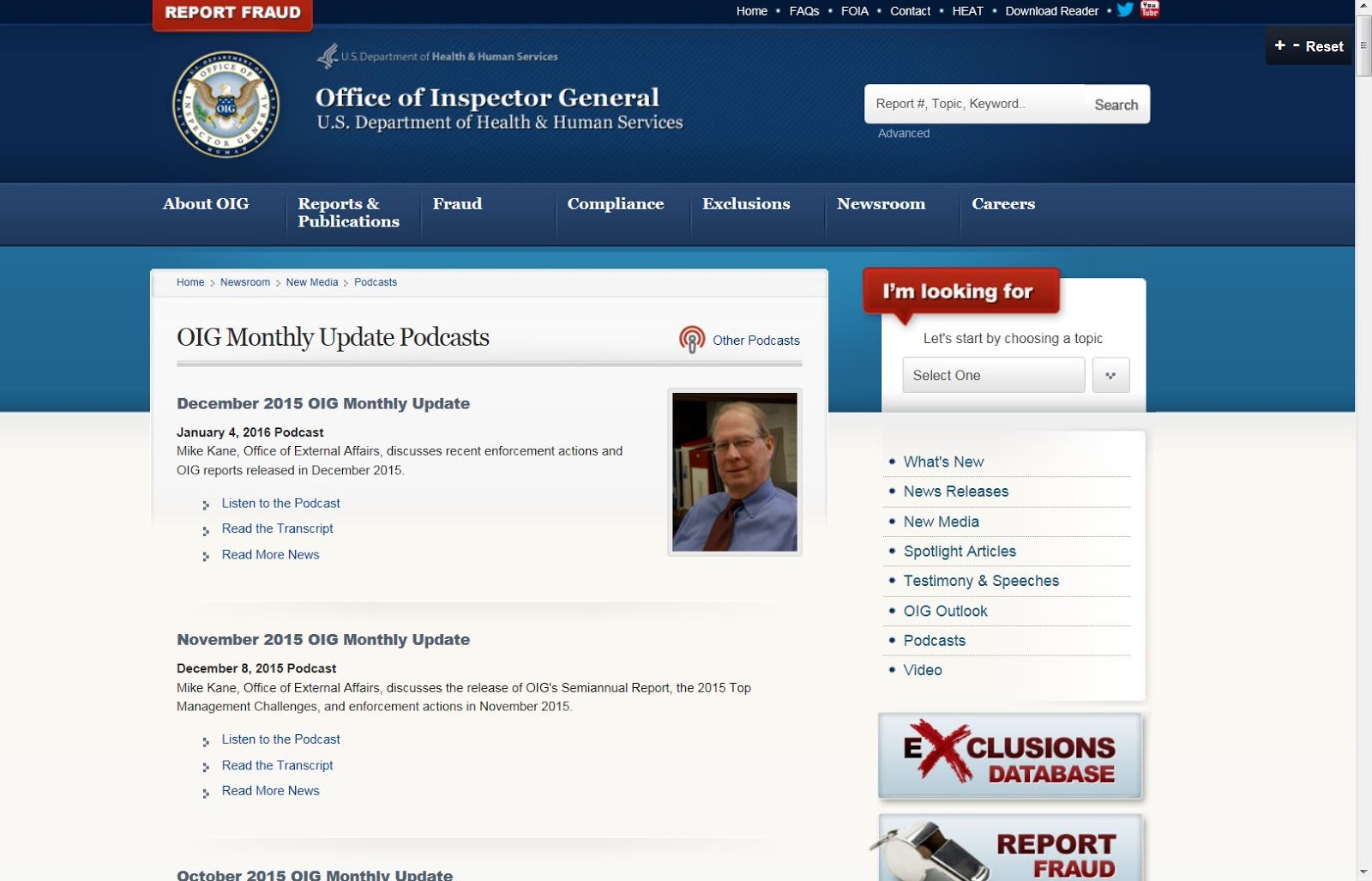The screenshot displays a webpage from the U.S. Department of Health and Human Services' Office of Inspector General. The page features a dark blue header transitioning into a lighter blue section, eventually giving way to a white lower section. Positioned on the top left, the phrase "Report Fraud" is prominently highlighted in red. Adjacent to this are drop-down menus labeled: Home, FAQs, Contact, Heat, and Download Features.

Centered within the dark blue bar is the round seal of the Office of Inspector General, followed by navigation links: About OIG, Reports and Publications, Fraud, Compliance, Exclusions, Newsroom, and Careers. Below this bar, a highlighted section reads "OIG Monthly Update Podcast," accompanied by a list of available episodes. Specific podcasts listed include the "November 2015 Monthly Update" and the "December 8, 2016 Podcast" featuring Mary Mae Cain from the Office of External Affairs.

To the right, there is a photograph of a middle-aged man wearing glasses and a necktie, with a receding hairline, adding a personal touch to the otherwise text-heavy layout.